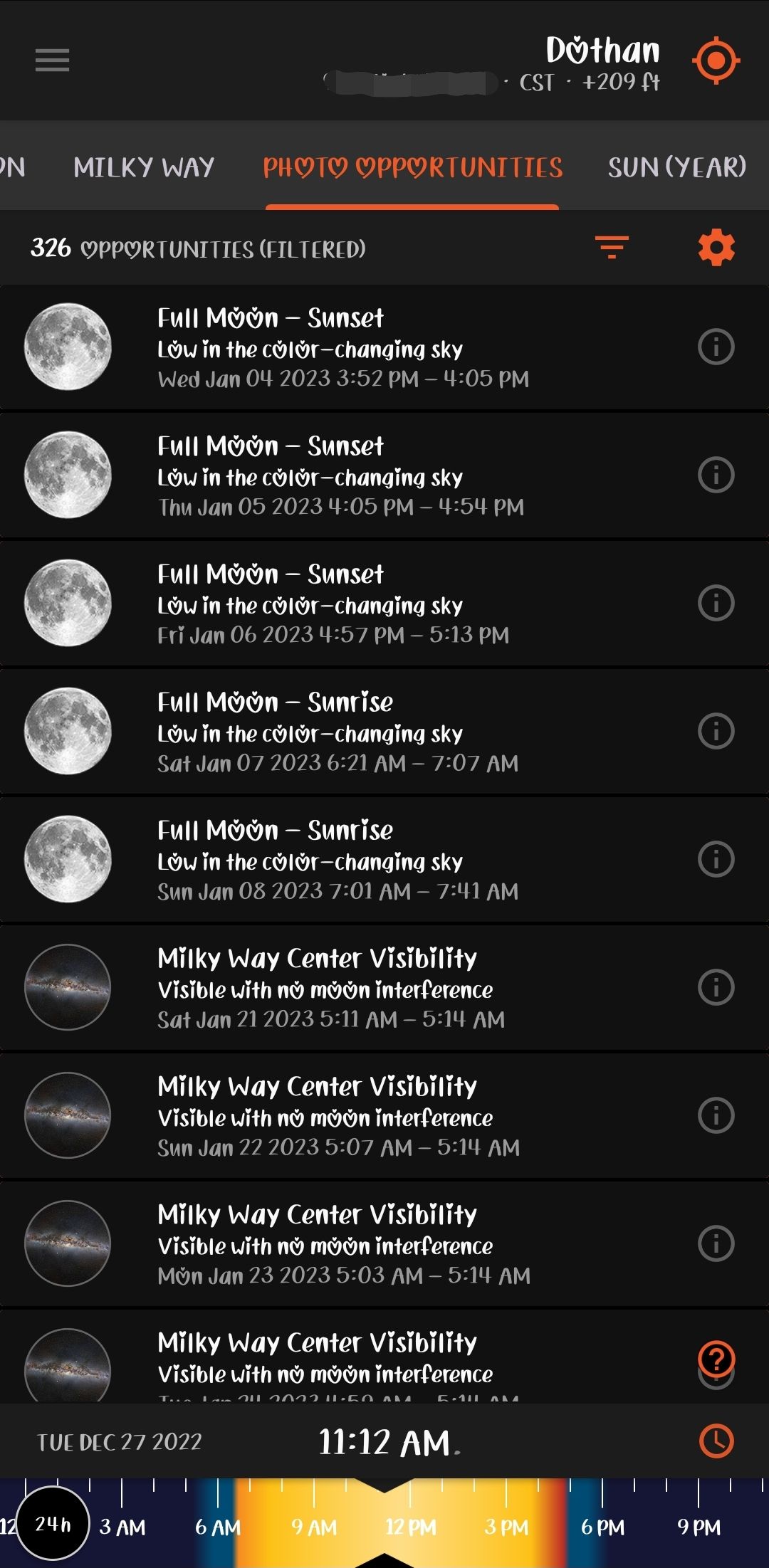A screenshot illustrating the interface of an app or program, possibly designed for stargazing or star tracking. The user interface exudes a sleek, modern feel with a predominantly black background, while the text appears in white and highlighted sections are marked in orange. At the top right corner, the display reads "Dothan," accompanied by a location icon, suggesting customizable location settings. Key details on the screen include references to "Milky Way visibility" and "sunset," hinting towards its utility in astronomy-related activities. One prominent section of the interface is the navigation bar, which lists "Milky Way" and "photo opportunities," with the latter being highlighted, indicating the active selection. Beneath the highlighted "photo opportunities" section are customized times, apparently showing the best periods to photograph the full moon, supporting the app's function as a tool for planning astrophotography sessions.